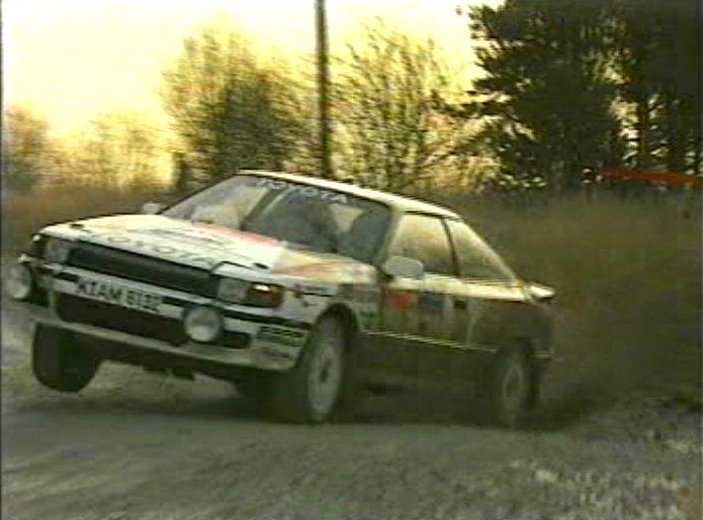A slightly blurry and aged photograph captures a Toyota rally car in an intense off-road race, barreling through a dusty, rocky path. The car, reminiscent of an older model Toyota Corolla or Celica, sports prominent "Toyota" decals on both the top of the windshield and the hood, with an array of other stickers and logos scattered across its dirty, predominantly white exterior. As the car maneuvers a tight turn, its rear wheels kick up a considerable cloud of dust, emphasizing its speed and the rough terrain. In the foreground, the front right wheel is momentarily suspended off the ground. The background features blurred trees and a large post, tinged with the warm, yellowish hues of the setting sun, enhancing the dramatic scene of a rugged, fast-paced rally event. The visible registration number, "KIAMB13," fades into the dusty, action-filled surroundings.